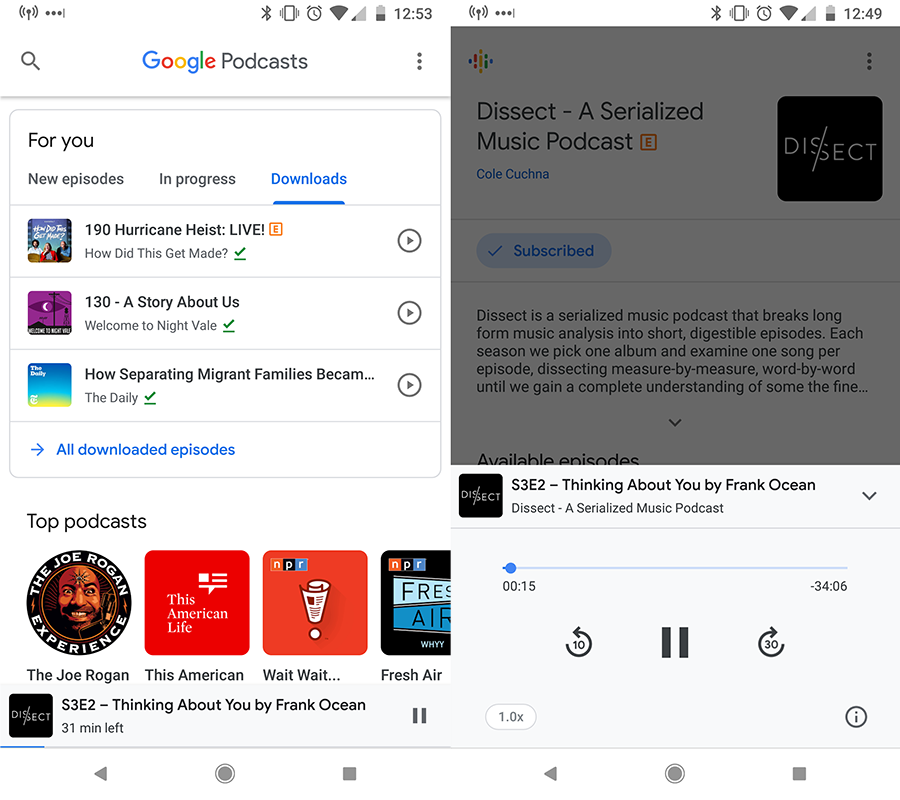The image consists of two screenshots showcasing different sections of the Google Podcasts interface. 

In the left screenshot, the header prominently displays "Google Podcasts." Below this, a navigation menu lists the sections: "For You," "New Episodes," "In Progress," and "Downloads." In the "Downloads" section, some notable entries are: "190 Hurricane Heist Live" from "How Did This Get Made" (with a duration of 1:30), "A Story About Us" from "Welcome to Night Vale," and the partially visible "How Separating Migrant Families Became..." from "The Daily." Following this, a list of "Top Podcasts" includes names like Joe Rogan, This American Life, Wait Wait... Don't Tell Me!, and Fresh Air.

The right screenshot reveals the now-playing screen, featuring the details of the podcast episode the person is currently listening to. Specifically, they are listening to "Thinking About You" by Frank Ocean, and they are 15 seconds into a 34-minute and 6-second episode. The playback controls show the main play button flanked by "Rewind 10 seconds" on the left and "Fast Forward 30 seconds" on the right. The time remaining is shown as "31 minutes left."